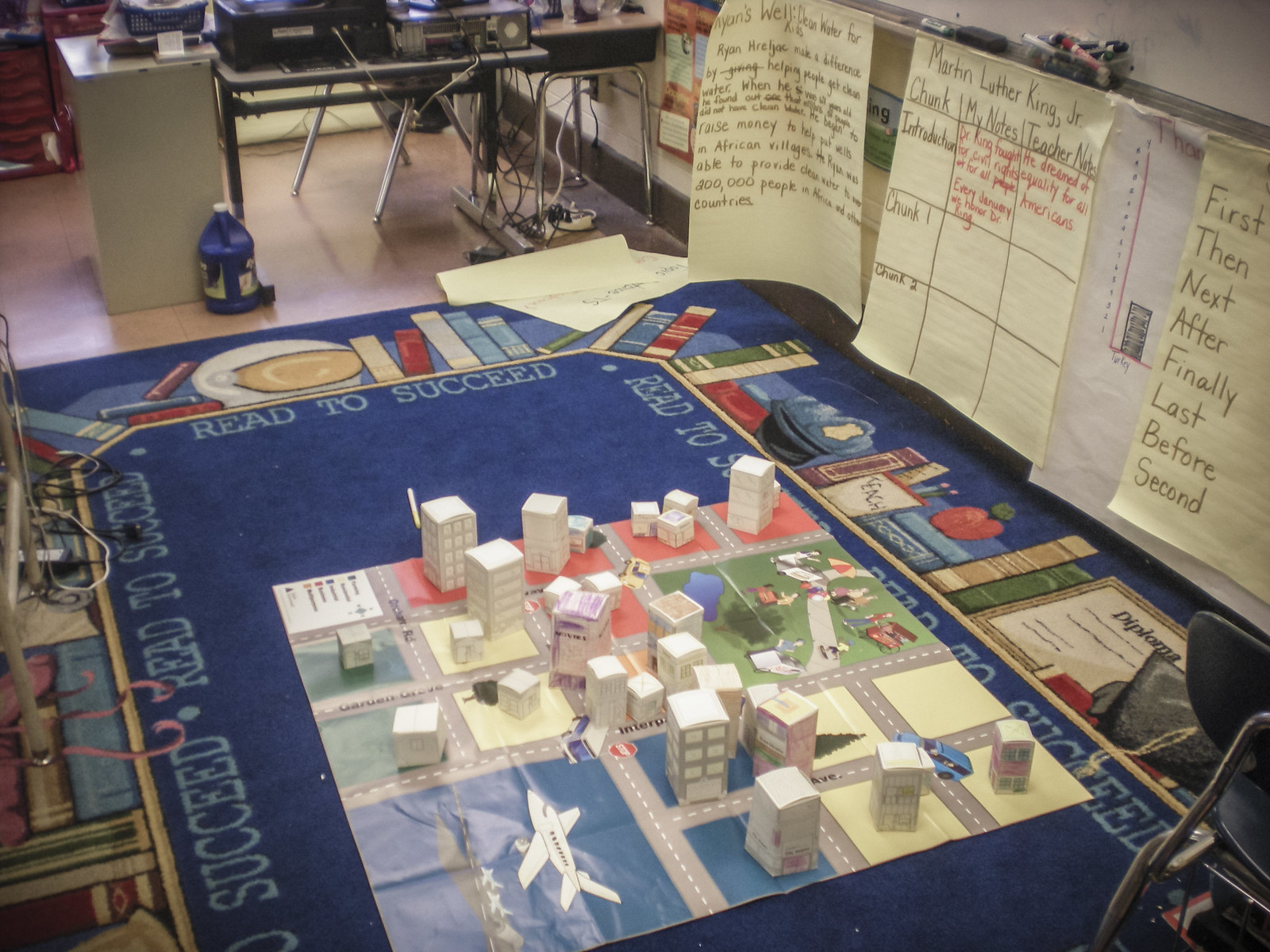This image features a detailed view of an elementary school classroom arranged for an engaging educational environment. In the top left corner, a teacher's desk is set up with a desktop computer and an assortment of cords connected to a power bar on the floor. A blue jug with a white cap sits on the ground beside a file cabinet, while light brown tiles cover the floor beneath.

Dominating the floor in the central area is a large, blue area rug bordered with the phrase "Read to Succeed," adorned with a bookshelf graphic. Centrally placed on this rug is a square playmat designed to resemble a cityscape, complete with roads, an airplane, and various buildings depicted. Rectangular objects resembling skyscrapers and other buildings are arranged on top of this playmat, likely used for teaching navigation skills.

On the upper right side, a bulletin board displays large sheets of paper. The middle sheet notably features the name Martin Luther King and is sectioned into parts with headings like "Introduction," "Chunk One," and "Chunk Two." This board serves as an educational tool, laying out brainstorming notes and teacher-directed content for students to reference during lessons.